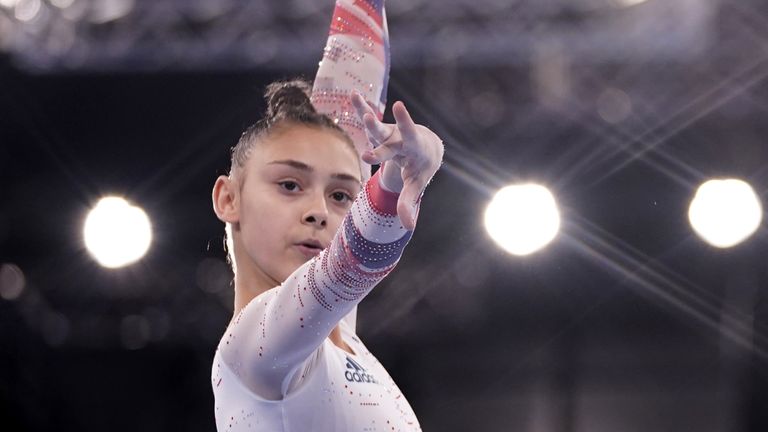This detailed photograph captures a gymnast in action, performing at a stadium. Positioned slightly to the left but occupying the full height of the image, she commands attention in her white leotard adorned with the Adidas logo in blue lettering on her chest. The leotard features red, white, and blue elements near the sleeves and hints of red and silver glitter-like dots. Her brown hair is neatly pulled into a bun atop her head, and she commands focus with a gesture—her middle finger tucked down, pointing towards the camera. The close-up reveals her tan complexion, suggesting she might be Hispanic, and her dedicated expression shows her deep engagement in gymnastics. The backdrop is a hazy stadium ceiling, with bright, out-of-focus lights and reflective steel girders providing an atmospheric setting for her performance.